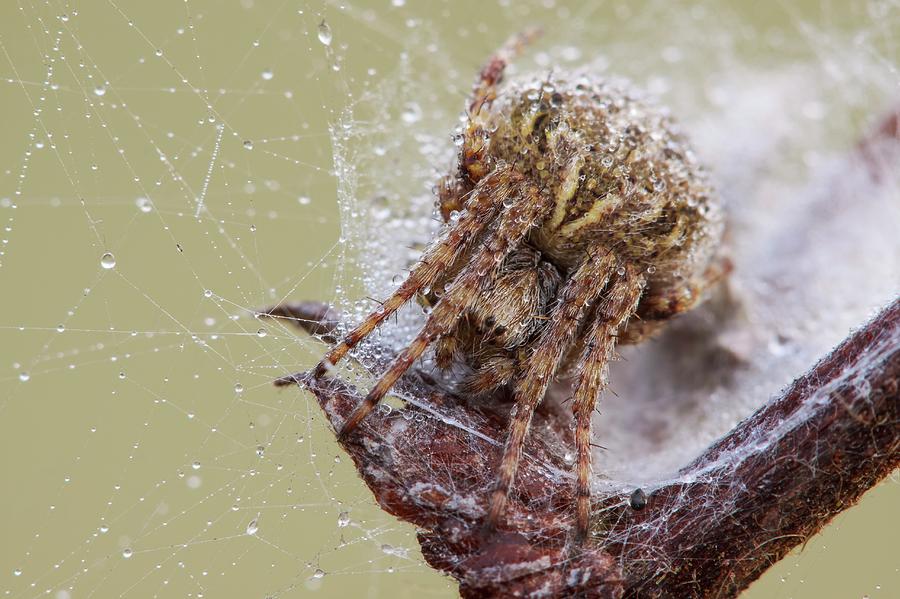The image depicts a close-up of a large, brown, and hairy spider with beige and brown markings. The spider, which has four legs visible and a distinct yellow V on its forehead, is perched in the crook of a tree branch covered in rough bark. The spider is surrounded by an intricate, white web that is geometric and densely woven in some areas, while appearing more random and looser in others. The web displays a noticeable sheen, likely from small water droplets, giving the spider and its surroundings a slightly wet appearance. The spider appears aged and is actively weaving the web around its position on the branch.